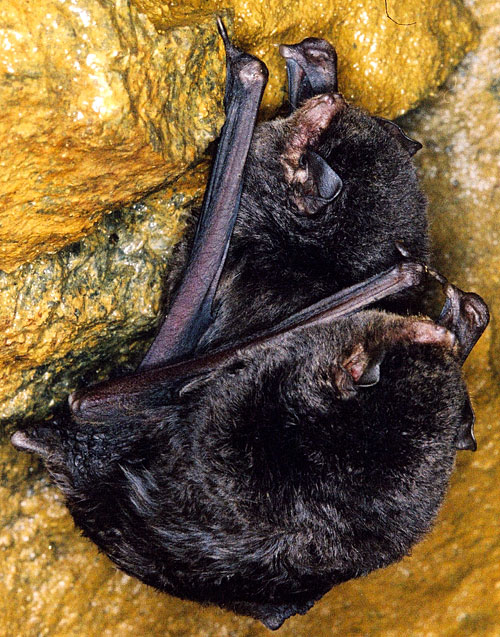The image is a close-up shot of two black bats with shiny fur, clinging to a wet, yellow, green, and beige-colored stone surface, giving the impression of a cave setting. One bat is positioned horizontally with its leg almost in front, while the other seems to be hanging upwards, possibly cleaning itself. They are resting closely together, using the hooks on their wings to grip the rock. The extreme close-up fills the frame with the bats, highlighting their black ears and wings as they nestle against the damp, detailed texture of the stone.